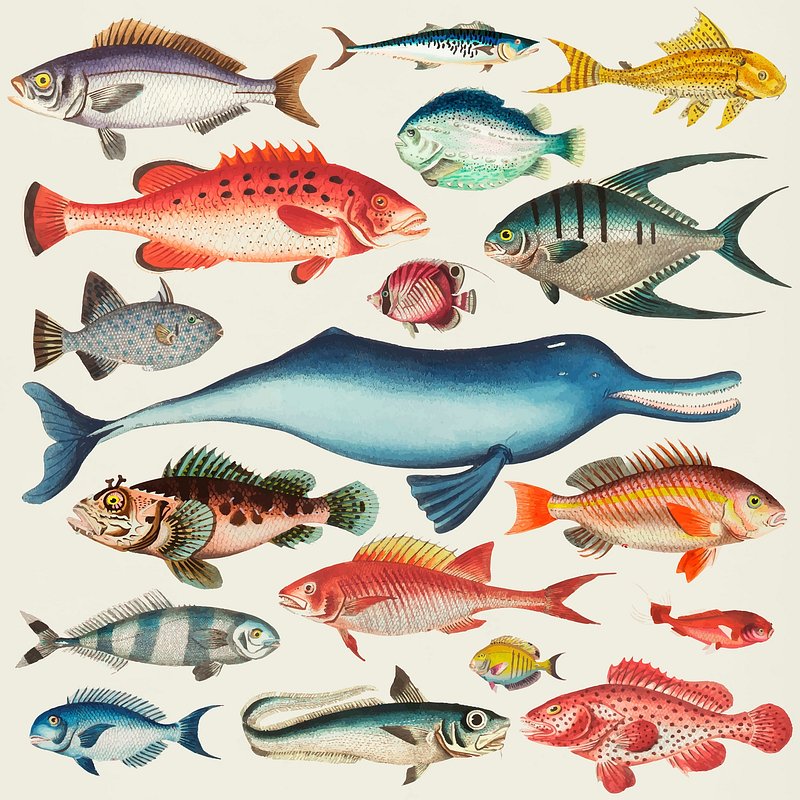This rectangular image, slightly taller than it is wide, depicts a visually rich art piece featuring 18 intricately detailed, colored pencil drawings of various fish and aquatic creatures against a cream background. The centerpiece is a striking, large creature with a long snout and numerous white teeth, reminiscent of a prehistoric dolphin or shark. Surrounding it are a multitude of freshwater fish, each uniquely patterned and vividly colored. The array of colors includes reds, oranges, blues, greens, purples, browns, grays, and metallic shades like green and yellow. Every fish is depicted with remarkable detail, showcasing their scales, fins, and tails, creating a vibrant and dynamic scene that would make a captivating decorative poster.